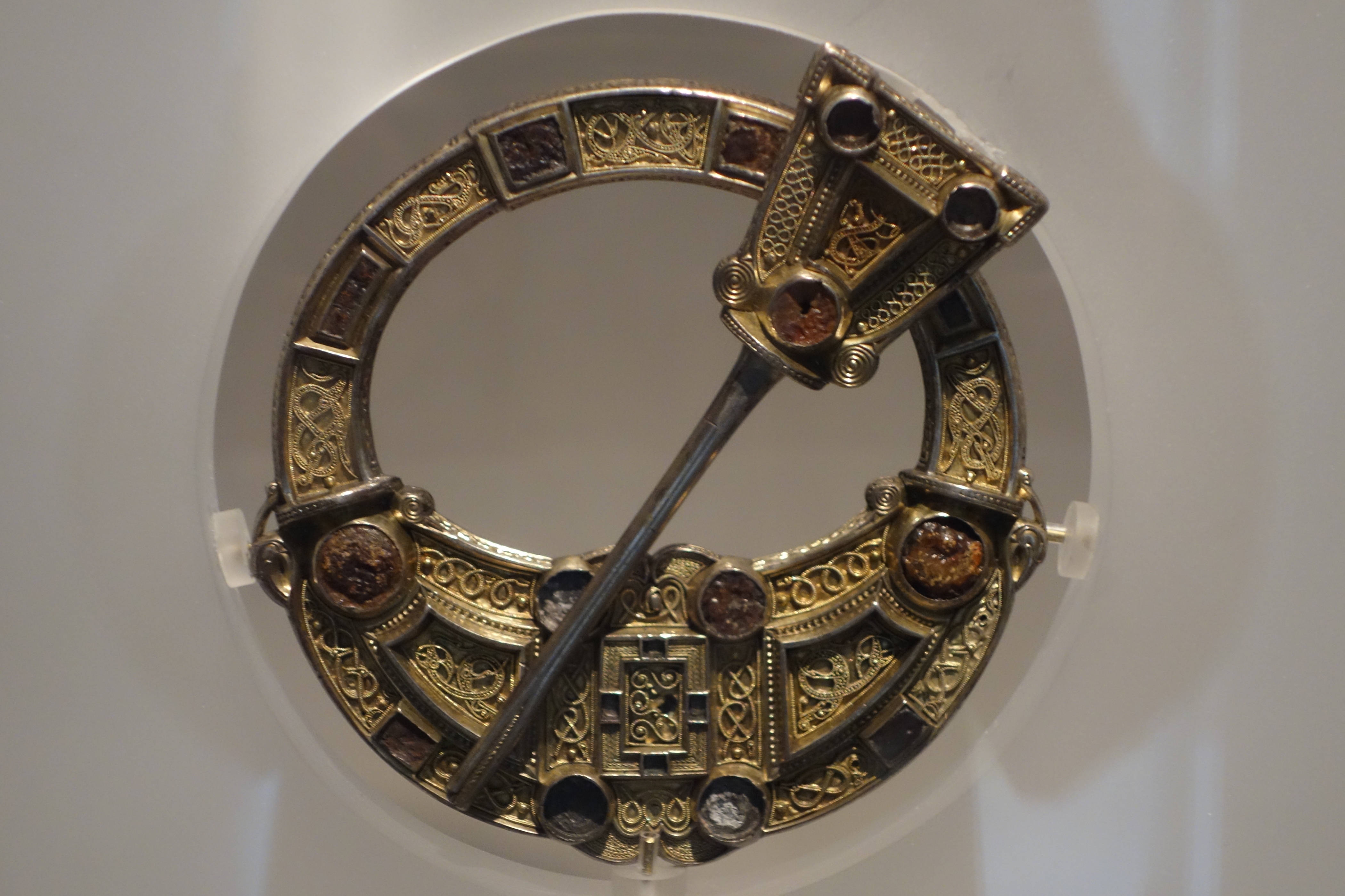This is a vivid color photograph showcasing a close-up view of an intricately designed, large circular ring. The ring appears to be crafted from a gold-like metal, possibly brass or actual gold, and is adorned with elaborate, beautiful embossing and ornate designs. Dominating the center, the ring features an oval-shaped front piece resembling a collar. Within this oval, there's an elaborate pattern that includes a central box surrounded by boxes on each of its four sides, forming a cross-like design superimposed with geometric shapes. Adding to the complexity, a thick, dull gray metal element diagonally intersects the design, reminiscent of a pen. At the top of the ring, a triangular motif mirrors the intricate patterns of the main body, adding a cohesive aesthetic to the overall design. The craftsmanship and elaborate details showcased in this close-up view highlight the ring's luxurious and artistic appeal.